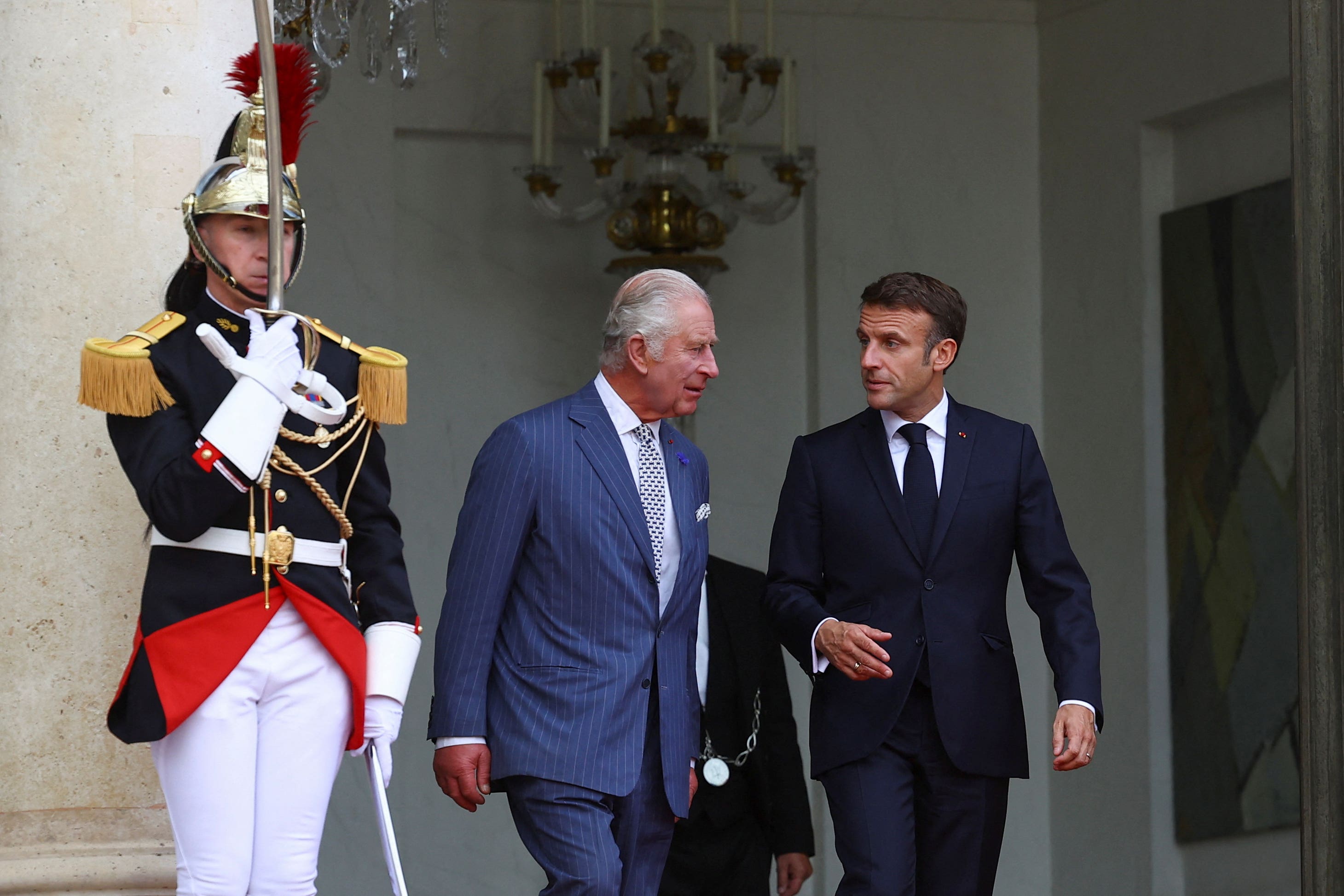In the photograph, King Charles III, distinguished by his gray hair and formal light blue suit with a white button-down shirt and a white tie with small black buttons, walks side by side with Emmanuel Macron, President of France. Macron is clad in a dark navy blue suit, complemented by a matching tie and a white button-down shirt. Both men appear to be engaged in conversation as they move forward. Flanking them to the left is a ceremonial guard standing at attention. The guard is wearing a gold helmet adorned with a red feather mohawk, a formal blue jacket with gold shoulder epaulets and tassels, a white belt, and tight white pants. He holds a sword vertically in front of his face. Behind them, there is a white wall with an elaborate chandelier featuring a gold vase design. The detailed regalia and formal attire make this a scene of distinguished political and ceremonial significance.